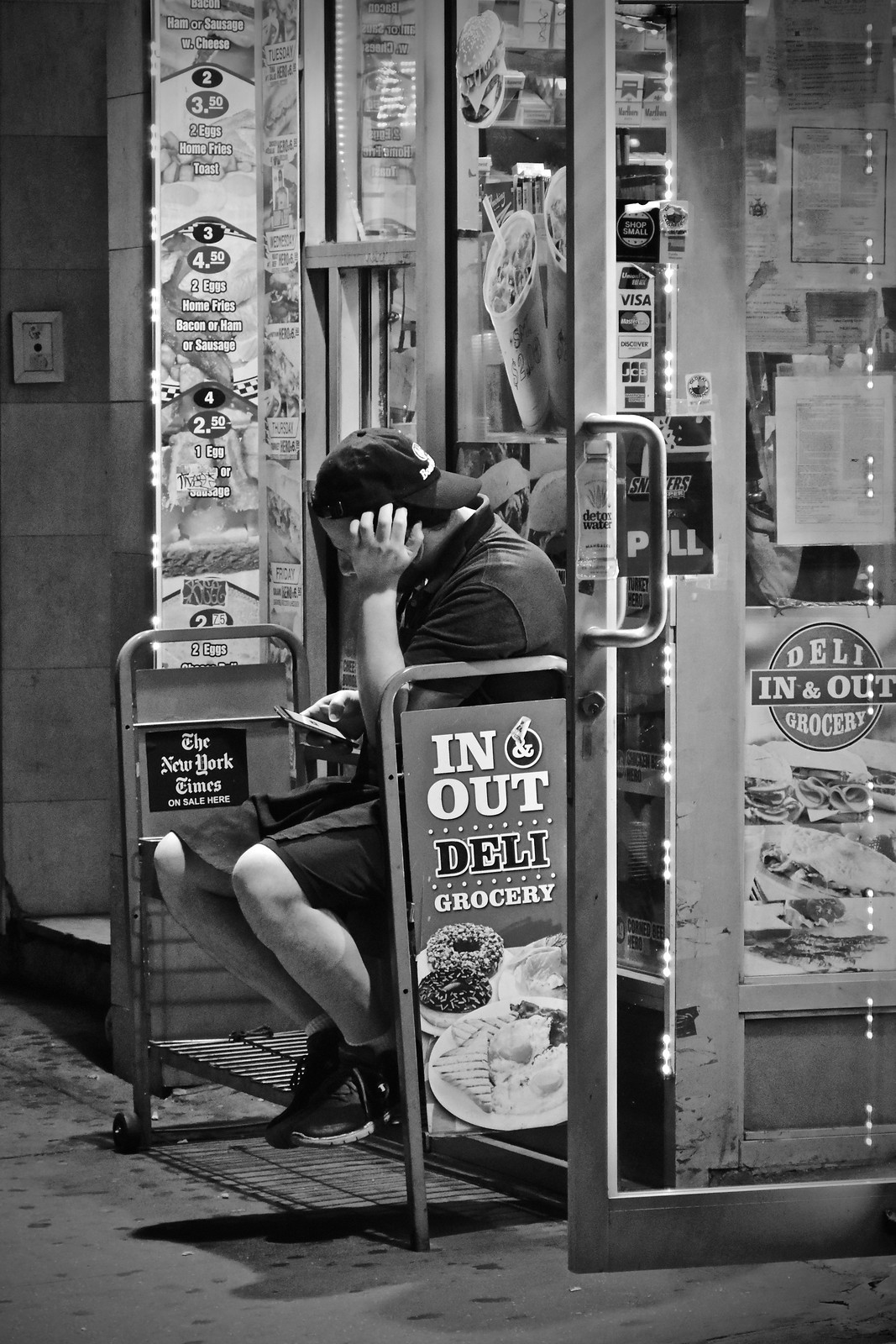This black-and-white photograph captures a scene outside the In-N-Out Deli and Grocery, likely in New York City. Centered in the image is a man seated on a bench, absorbed in his phone. He is dressed in black tennis shoes, black shorts, a dark shirt, and a backwards dark baseball cap. His left arm supports his head, shielding his face from view. The bench stretches to his right and left, while a concrete floor occupies the bottom fourth of the image. 

To his right, an open door leads into the deli, and above him, windows display multiple advertisements. Signs visible in the image read "In-N-Out," "Deli," "Grocery," "Visa," "MasterCard," "Discover," and "The New York Times on sale here." Additional signs offer specials such as "Two eggs, home fries, bacon, or ham or sausage for $4.50" and "Ham or sausage with cheese for $2." Other visible advertisements feature images of donuts, toast, fried eggs, bacon, milkshakes, soft drinks, pizza, and "detox water," along with a "Snickers" sign.

The photograph, executed with great attention to detail, evokes a sense of a casual, everyday moment, with the man seemingly taking a break outside the busy deli.